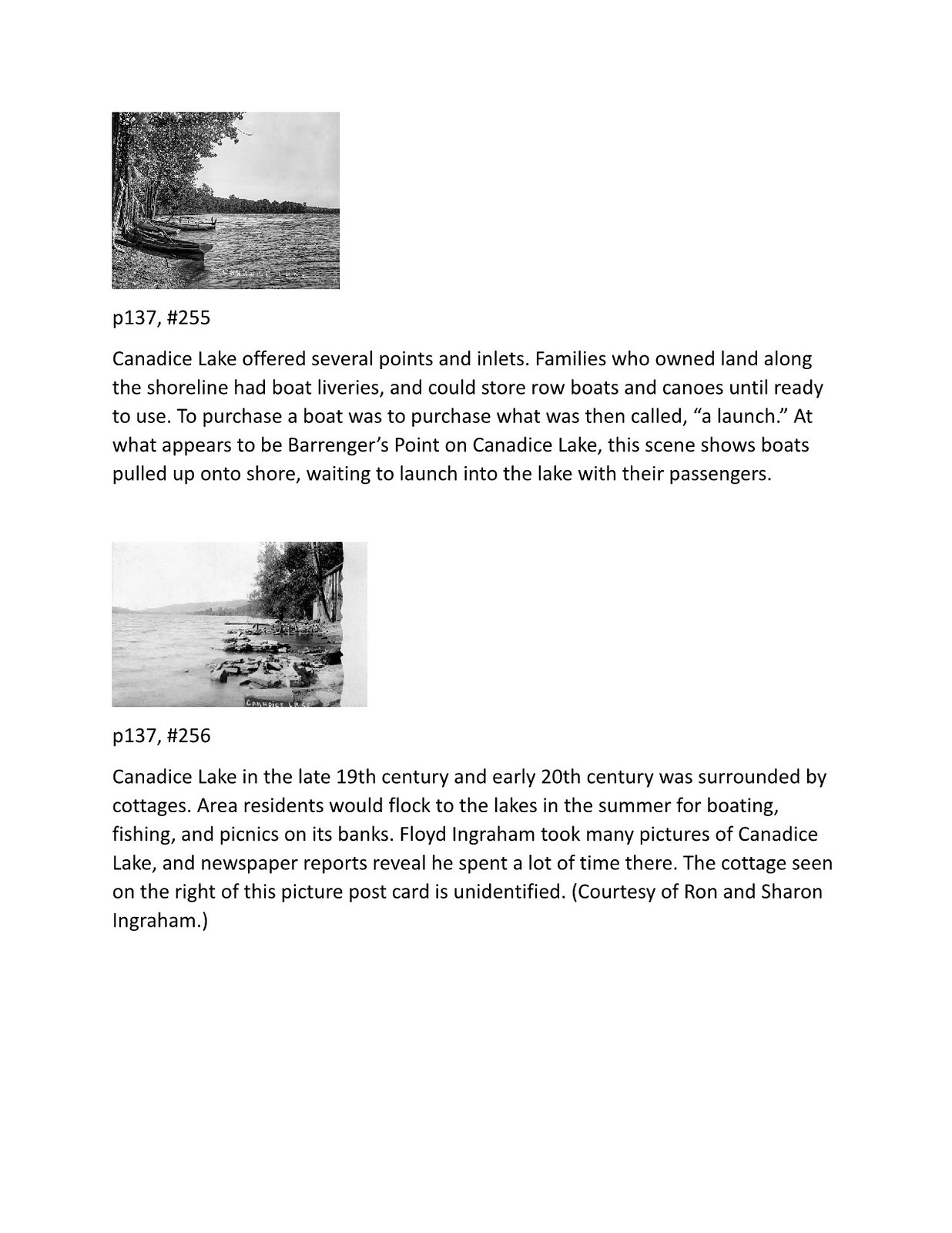On a white background, there are two small black and white photographs positioned one above the other. The top left photo depicts a lake with a riverbed to its left and various canoes and rowboats pulled up onto the shore, with numerous trees lining the bank. The sky is visible. Under this image, there is a text identifier that reads "Page 137, #255." Adjacent to this photograph is a paragraph explaining that this is Candice (Canada's) Lake, which offers several ponds and inlets. Historically, families who owned land along the shore had boat liveries where they could store rowboats and canoes until they were ready to be used. The paragraph details that to purchase a boat at that time was to buy what was known as a launch. At what appears to be Baronga's (Baringers) Point on Candice Lake, the scene shows boats awaiting launch into the lake with their passengers. 

Below this, there is another black and white photograph of a lake or river, flanked by a wall and some trees on the right side. It is similarly labeled with "Page 137, #256." This accompanying paragraph provides historical context, noting that Candice Lake was surrounded by cottages in the 19th and early 20th centuries. Local residents would visit the lake in the summer for boating, fishing, and picnics. The image is credited to Lloyd Ingraham, a photographer who captured many scenes of Candice Lake, with newspaper reports indicating his frequent visits to the area. The postcard contains an unidentified cottage scene on the right, courtesy of Ron and Sharon Ingraham.